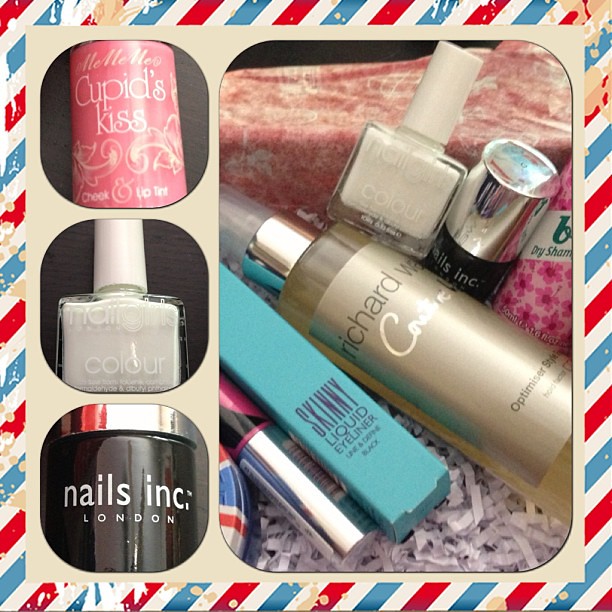The image showcases a single box framed by a tarnished red, white, and blue border resembling a barber pole, with paint splashes scattered across it. Within the box, the contents are divided into four sections: three vertically stacked images on the left and one large image on the right. In the top left photo, there is a product labeled "Cupid's Kiss Cheek Uptint" in a bottle. The middle image displays a white nail polish named "Nail Girl's Color." The bottom left features a "Nails Inc. London" black jar with a silver cap. The large image on the right side highlights an array of beauty products scattered over paper confetti, including "Skinny Liquid Eyeliner," and several items from the "Nails Inc." brand. The products' labels visible in the image include "Cupid's Kiss," "Nails Inc.," and "Skinny Liquid Eyeliner." The colors present in the image are red, white, blue, tan, pink, black, gray, light blue, and silver. This detailed composition suggests the image's purpose is to showcase a variety of makeup and beauty products.